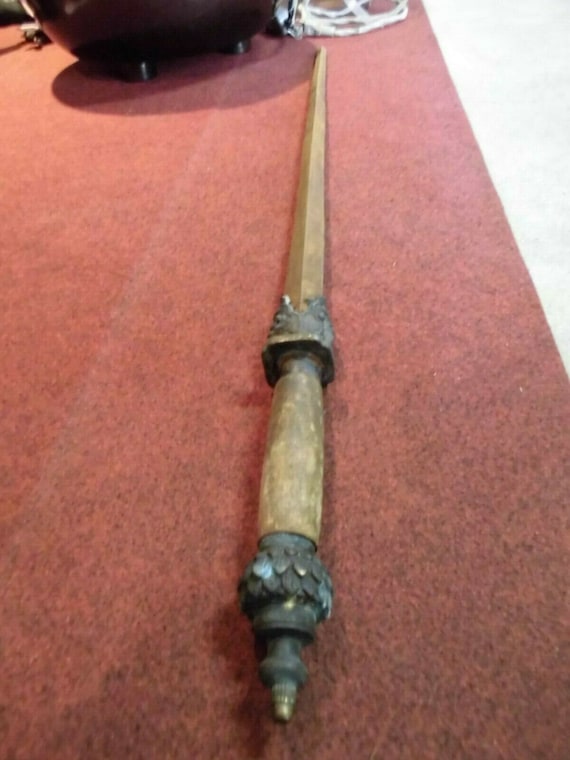The image depicts a finely crafted wooden sword, likely medieval-inspired, resting on a grainy red rug. The sword, which might be a type of practice or costume piece, features intricate carvings on the handle, resembling feathers. Both the handle guard and the decorative end cap appear to be made of weathered bronze or brass. Metal braces are also visible near the bottom and about a foot up the wooden blade. The sword's smooth handle is positioned in the foreground, while the tip extends into the distance. The upper right corner of the image reveals a glimpse of a white floor, and a circular object with feet is partially visible in the top left, just beyond the wooden sword.